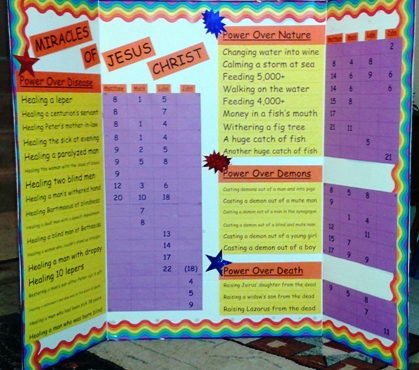The image depicts a vividly colorful school project display board titled "Miracles of Jesus Christ," bordered by a prominent rainbow design. The tri-fold board measures approximately 3 feet tall by 4 feet wide, featuring a larger central panel flanked by two smaller side panels. Each miracle is categorized into sections with color-coded tables, predominantly purple, which are sometimes difficult to read due to their size. 

Highlighted sections include "Power Over Disease," listing miracles such as healing a leper, healing ten lepers, and healing a centurion's servant. Another section, "Power Over Nature," details events such as changing water into wine, calming a storm, feeding 5,000, walking on water, and finding money in a fish’s mouth. "Power Over Demons" features miracles like casting a demon out of a boy. "Power Over Death" rounds out the categories, though the specific miracles in this section are too small to decipher.

The board is not only informative but visually engaging, with a red background for the titles, purple tables framing the text, and yellow listings for the different events. Small illustrated elements such as blue splat designs add to the dynamic and engaging presentation, making it an eye-catching project likely intended for a science fair or religious study showcase.